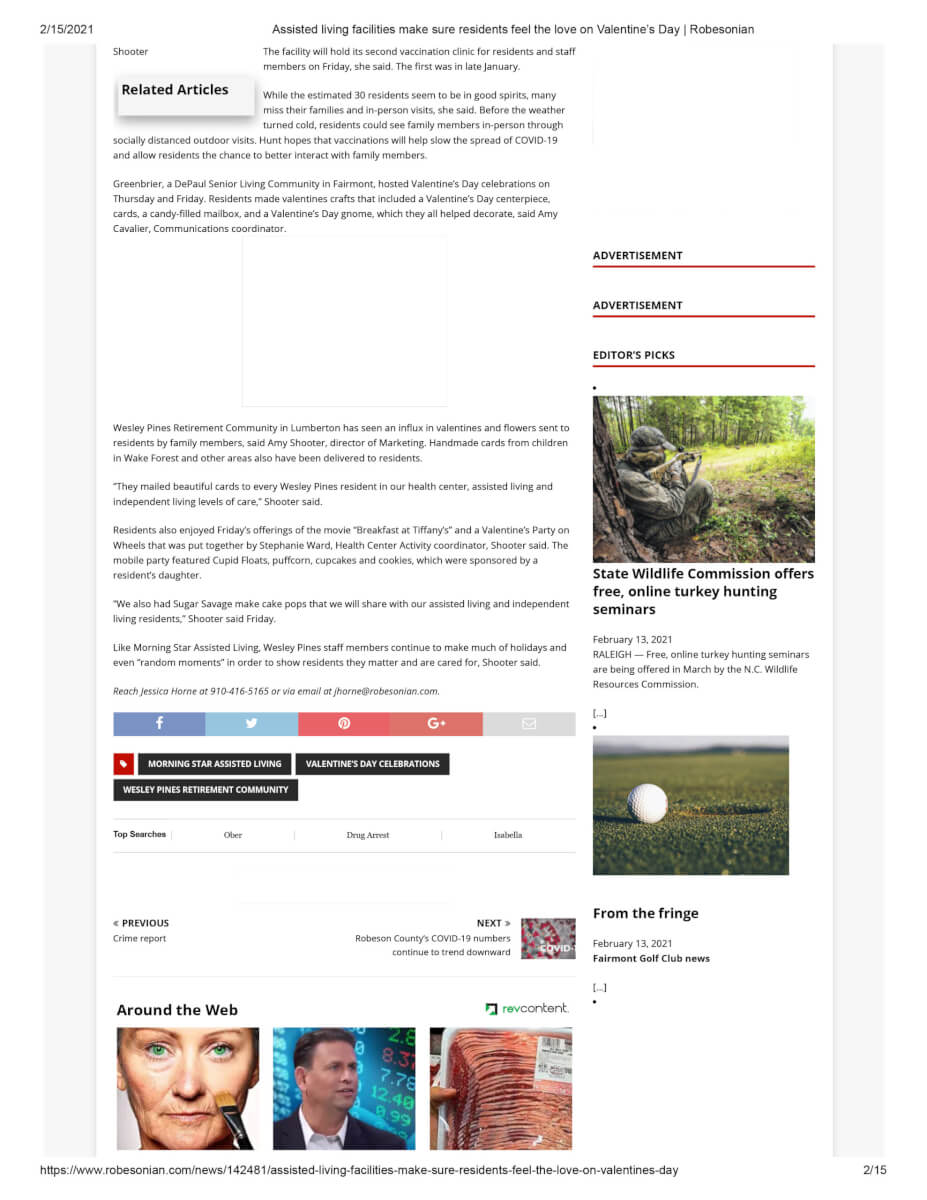**Caption:**
  
On February 15, 2021, an article written by Robesian highlighted the heartwarming Valentine's Day celebrations organized by several assisted living facilities to ensure residents felt cherished during the holiday. The article, titled "Assisted Living Facilities Make Sure Residents Feel the Love on Valentine's Day," detailed the efforts of Greenbrier, a DePaul senior living community in Fairmont, and Wesley Pines Retirement Community in Lubberton.

At Greenbrier, residents engaged in crafting activities, creating Valentine's Day centerpieces, cards, a candy-filled mailbox, and even a festive Valentine's gnome. Amy Cavalier, the communications coordinator, mentioned that these activities were held on the Thursday and Friday preceding Valentine's Day.

Wesley Pines Retirement Community saw a generous influx of Valentine's cards and flowers from family members. Amy Schueter, director of marketing, highlighted that handmade cards from children in Wake Forest and other areas were also delivered to the residents. Schueter shared details about a special offering of the movie "Breakfast at Tiffany's" and a unique Valentine's party on wheels, which featured Cupid floats, puff corn, cupcakes, and cookies, thanks to the sponsorship of a resident's daughter. Stephanie Ward, the health center activity coordinator, organized this mobile party. Additionally, a Sugar Sauvage cake pops treat was shared with both assisted living and independent living residents.

The article also noted that staff members at Wesley Pines and Morning Star Assisted Living strive to make holidays and everyday moments special for their residents. Social media links, an email option, and comment sections were provided at the bottom of the article page, which also contained various advertisements.